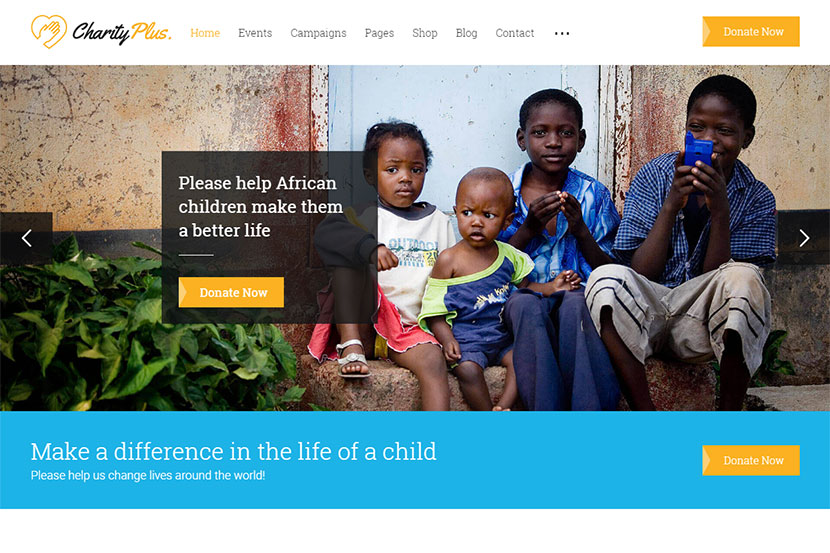In the web page image for CharityPlus, the primary navigation links are arranged prominently at the top, showcasing options including Home, Events, Campaigns, Pages, Shop, Blog, Contacts, and a conspicuous "Donate Now" button. The page features a strong call-to-action headline: "Please Help African Children – Make their Lives Better by Donating Now." This is followed by an inspiring subtext: "Make a Difference in the Life of a Child – Help Us Change Lives Around the World."

The color scheme of the web page is cohesive, incorporating black, yellow, white, and blue, which provides a visually appealing and professional look. In the background, there is a poignant image of six children. Four of the children are captured with joyful, smiling faces, radiating happiness and hope. In contrast, two other children exhibit indifferent expressions, presenting a more somber and contemplative mood. All the children appear well-nourished and healthy, symbolizing the positive impact of contributions and support provided through the charity.